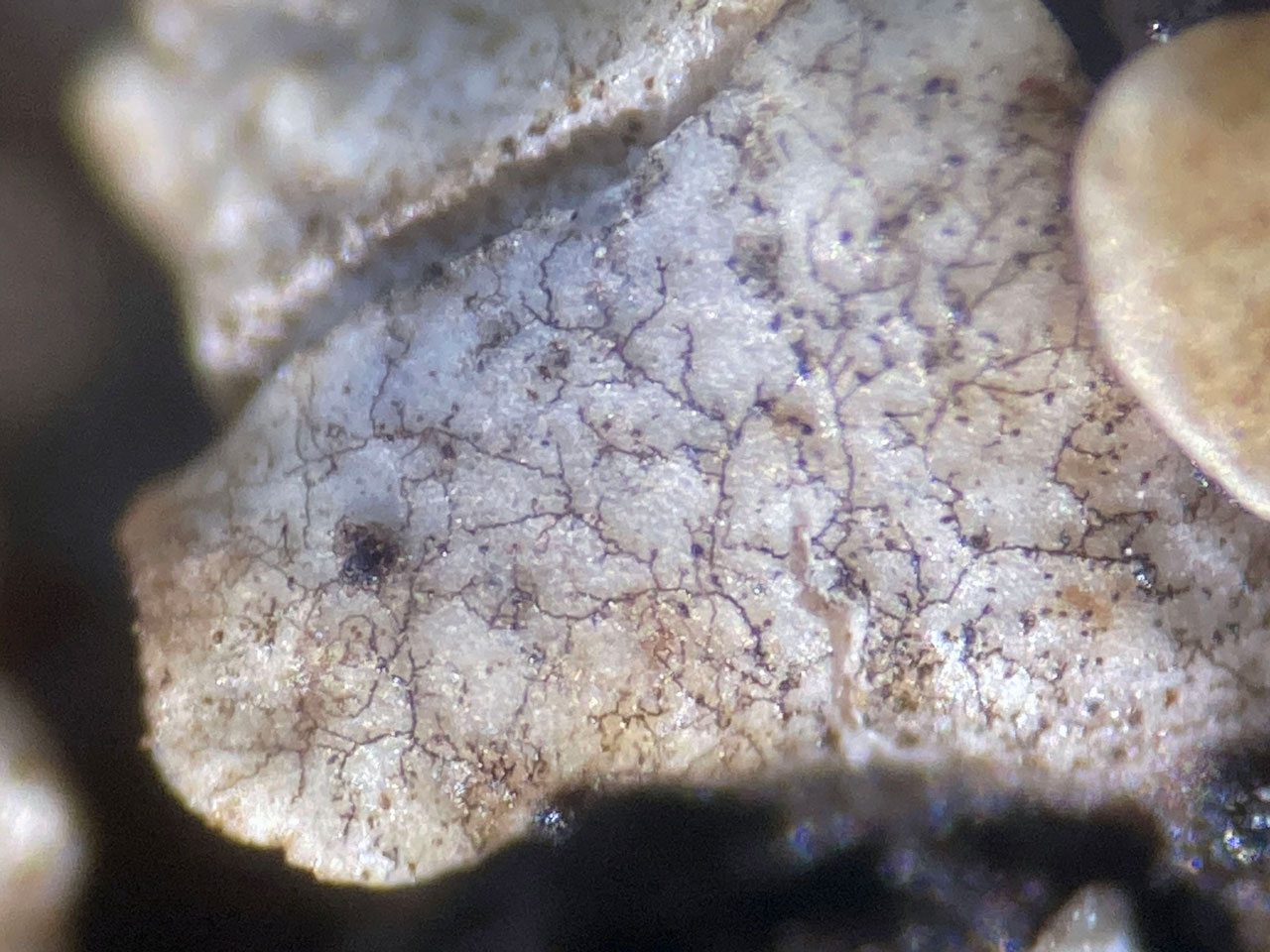This image showcases a close-up of a jagged, triangular-shaped rock formation, predominantly gray-beige in color with intricate thin veins running through it. The rock's surface is interspersed with fine black and blue vein-like lines that stretch across its entire expanse. Its texture, somewhat resembling sugar cubes, is set against a stark black background. Toward the bottom right, a shine gives a hint of blackness against the grainy surface. Additionally, in the top right corner, there appears to be another blurry, spherical object with a beige hue, partially covering part of the rock and its surrounding area. The overall shape of the rock evokes an organic and uneven form, with some edges appearing blurred.